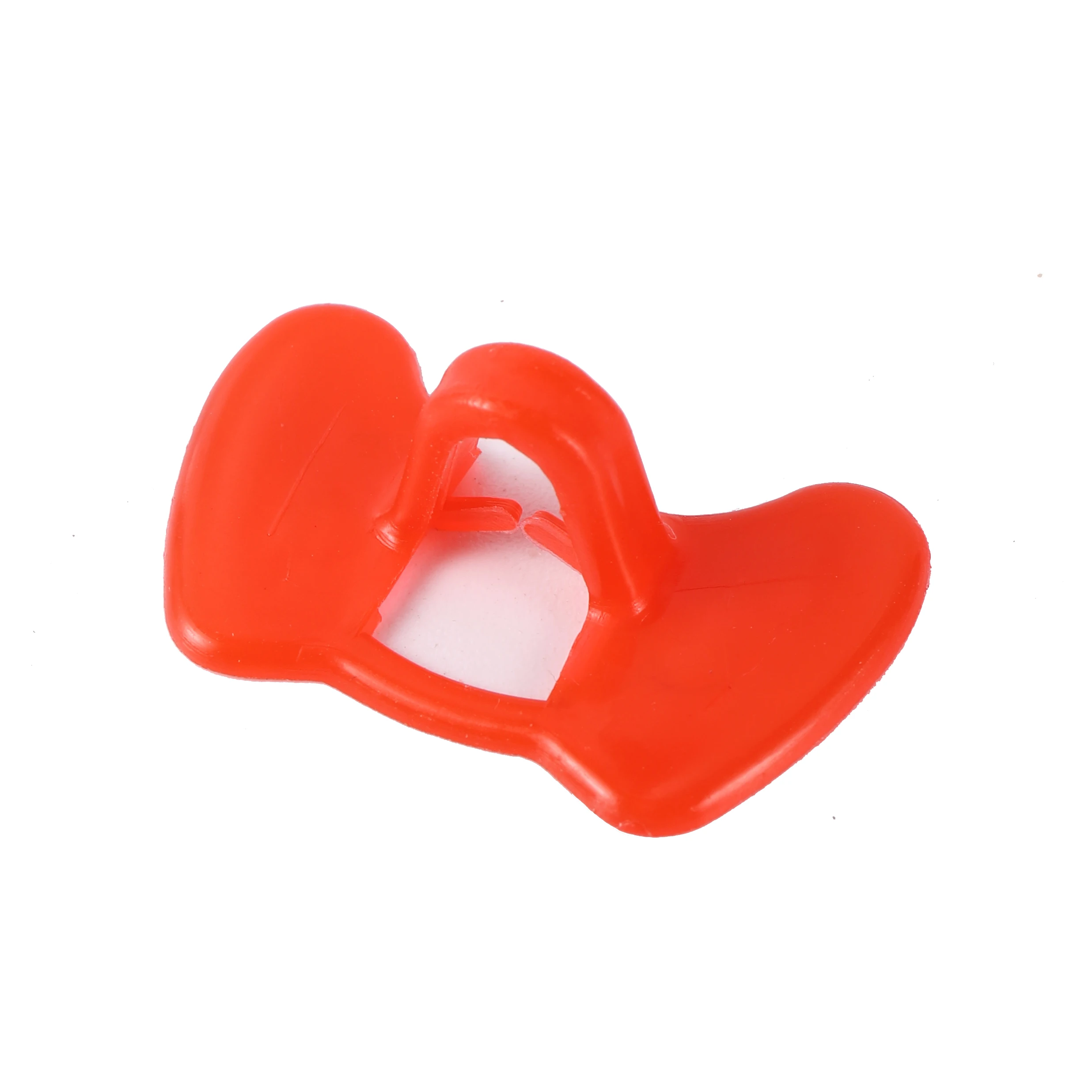This image features an orange, plastic object set against a solid white background. The object resembles a baby's pacifier but with unique design elements. It has two oval pieces resembling human lungs, positioned on either side, likely to prevent swallowing. These lung-shaped parts are connected by a V-shaped orange rubber piece, designed to fit inside the baby's mouth. Below this V-shaped rubber piece, there are two smaller, unconnected pieces of orange rubber. An additional lower band connects the lung-shaped sections, ensuring structural integrity. The overall design, highlighted by its reddish-orange color and plastic material, appears to be a blend of functional and unique aesthetics, somewhat reminiscent of chicken glasses or a bow tie.